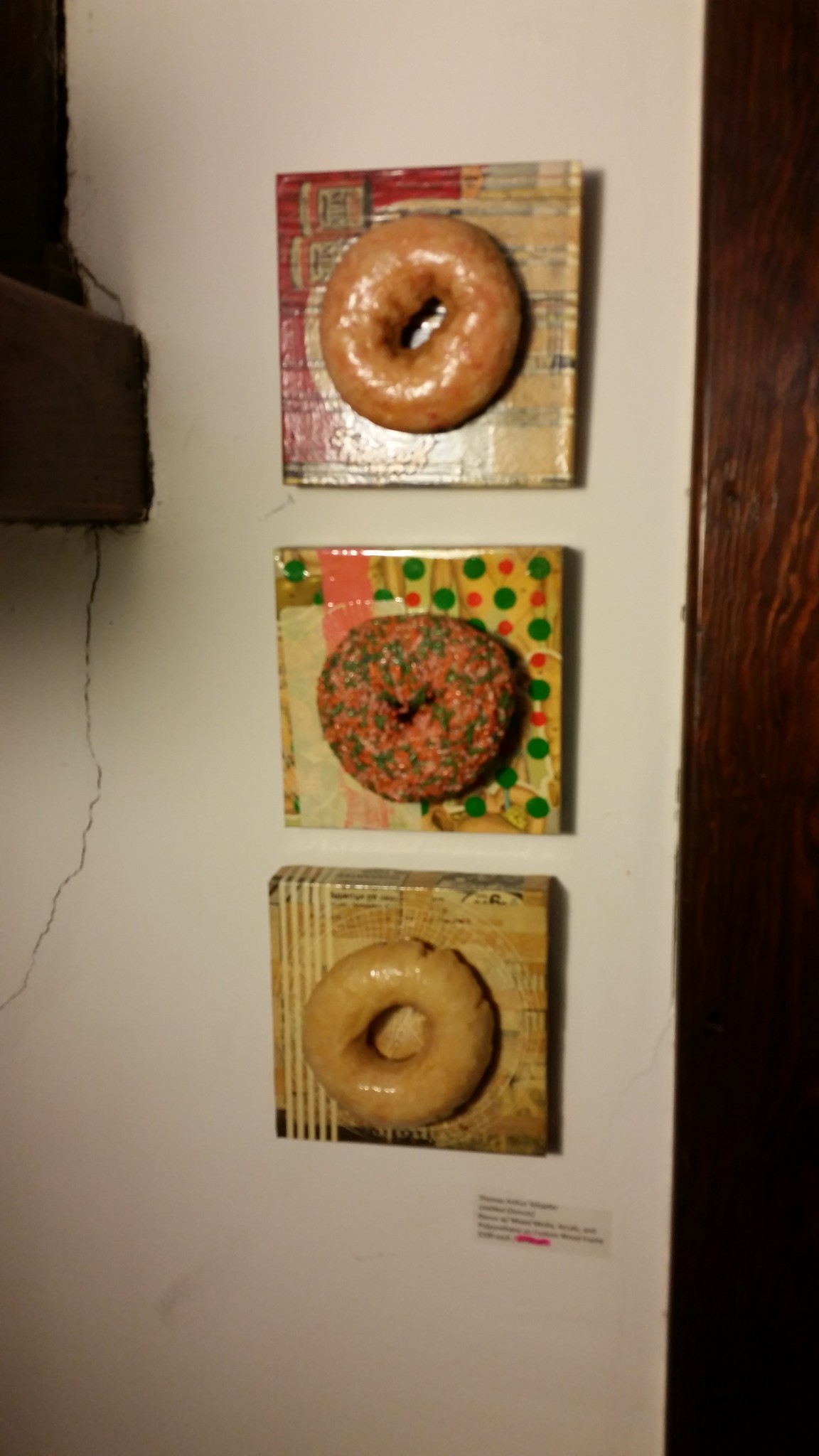The photo captures three doughnut-themed plaques arranged vertically on a white interior wall. The composition is slightly blurred, and the wall exhibits signs of age with visible staining and a prominent crack extending downward from a shadowy shape in the upper left of the image, potentially a window stool. On the right side of the photograph, a piece of dark wooden trim extends up and down, characterized by its visible grain, hinting at the old age of the setting.

The three plaques each feature a three-dimensional doughnut set against vibrant, decoupaged backgrounds. The top plaque displays a glazed doughnut on a background with red and tan hues. The middle plaque showcases a doughnut adorned with colorful sprinkles in shades of green, pink, and yellow, set against a background with a tan and dotted pattern. The bottom plaque contains a plain doughnut with another tan and patterned background. Below this plaque, there is a small piece of paper with some text, although it is not legible in the photograph.